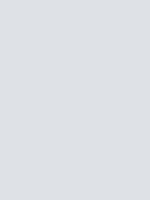This image appears to be a placeholder, indicating that the actual content did not load. It consists of a large, solid, light gray rectangular box occupying the space where the image should be. The box is devoid of any objects, text, or intricate details, serving purely as an empty placeholder. It suggests that the intended image is missing or failed to load due to some error on the website.